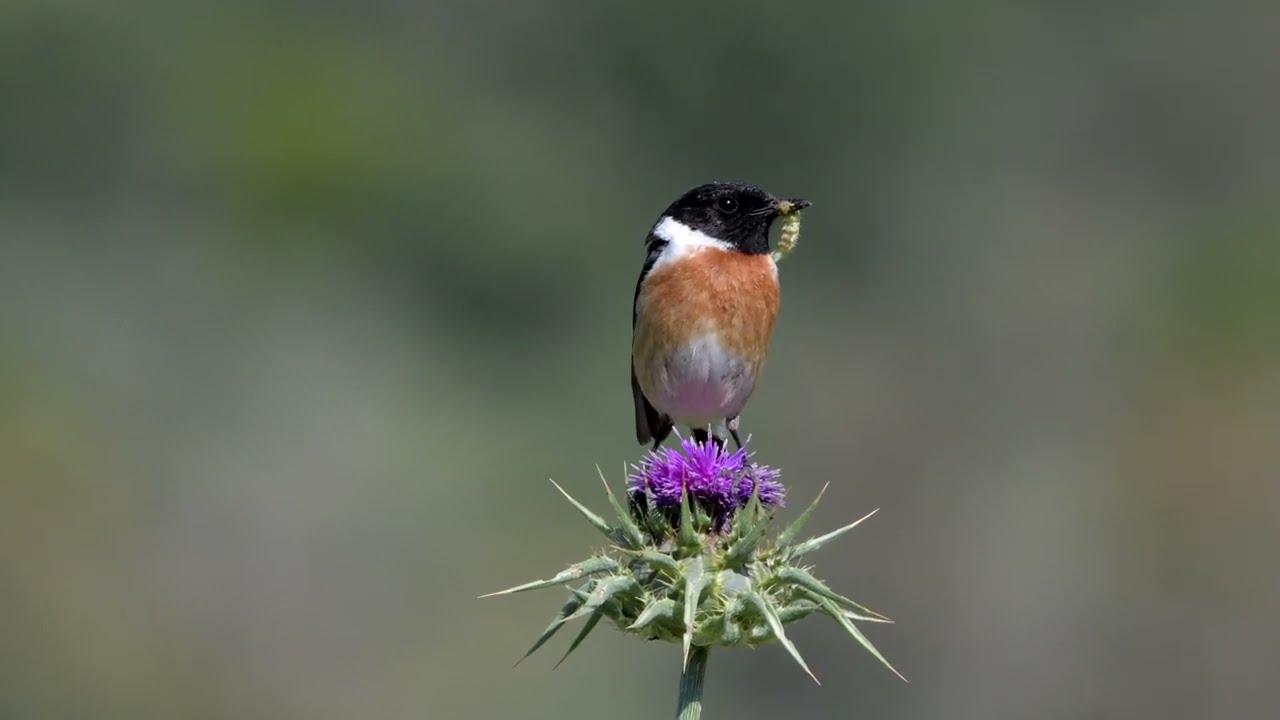In the foreground of this detailed color photograph, a tiny bird perches atop a purple flower. The flower is supported by a long stem and is surrounded by numerous green thorns that fan out from its base. The bird, with its back to the viewer, is the center of attention. Its head is turned slightly to the right, showcasing a black head adorned with a white ring around its neck. The bird boasts a reddish-brown chest that transitions into white underneath, and its folded wings are a stark black. A small insect dangles from its black beak, which is marked with a white splotch. The background is an out-of-focus gray-green, keeping the focus sharply on the bird and the flower. The photograph captures the intricate details of the bird’s feathers and the spiky structure of the plant, presenting a vivid example of photographic representational realism in a landscape orientation.